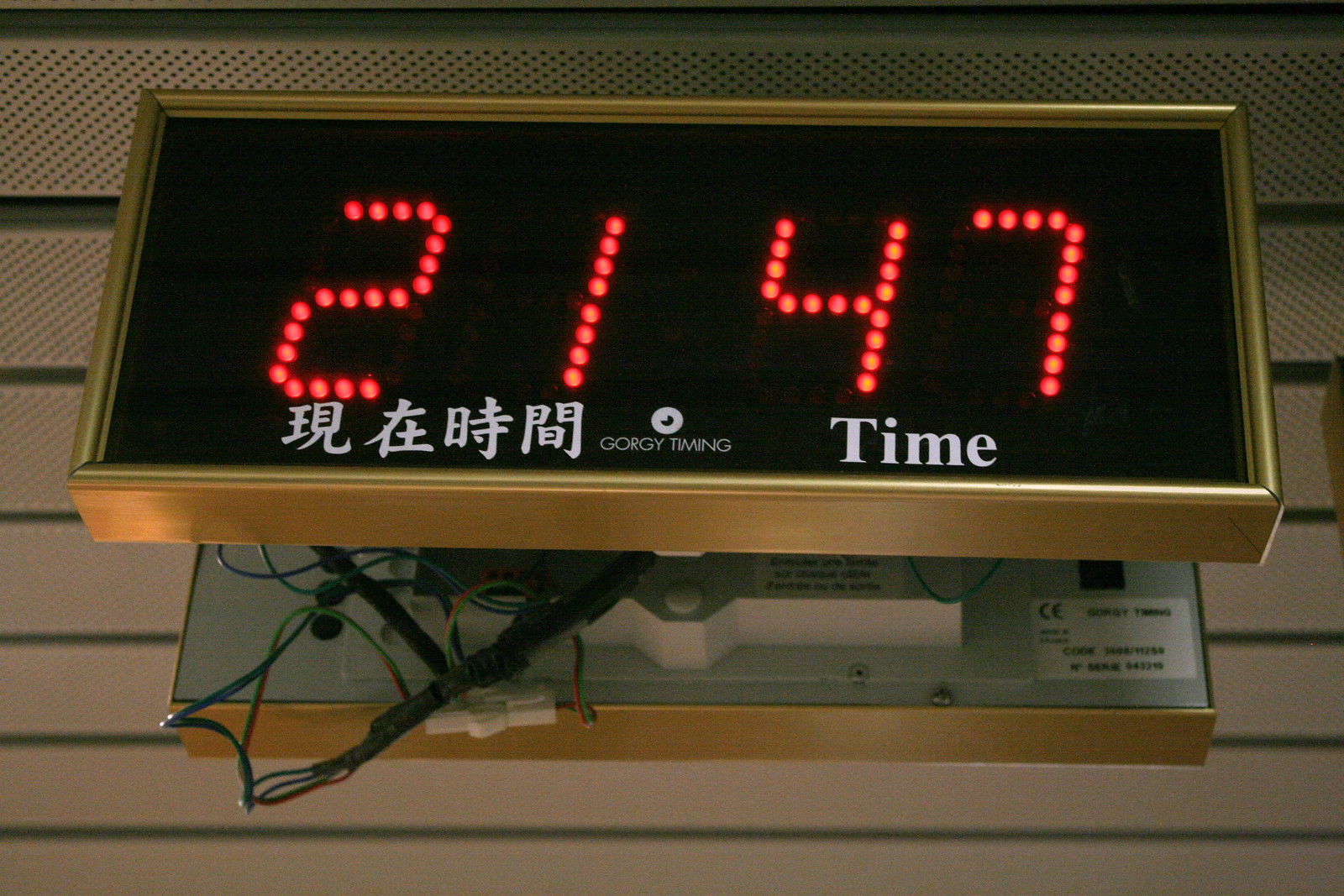In this photograph, the background features a ceiling or wall composed of beige-painted metal panels, each with numerous circular perforations. Suspended from this ceiling is a rectangular digital clock. The clock has a golden metal frame surrounding a black display. The display showcases red LED numbers, indicating the time as '21:47.' Below the '21,' there is some Asian writing, while the word 'corgi twinge' appears in the center of the display. Below the '47,' the word 'time' is shown in white font. The intricate detailing of the ceiling and the vibrant digital clock create a striking contrast.